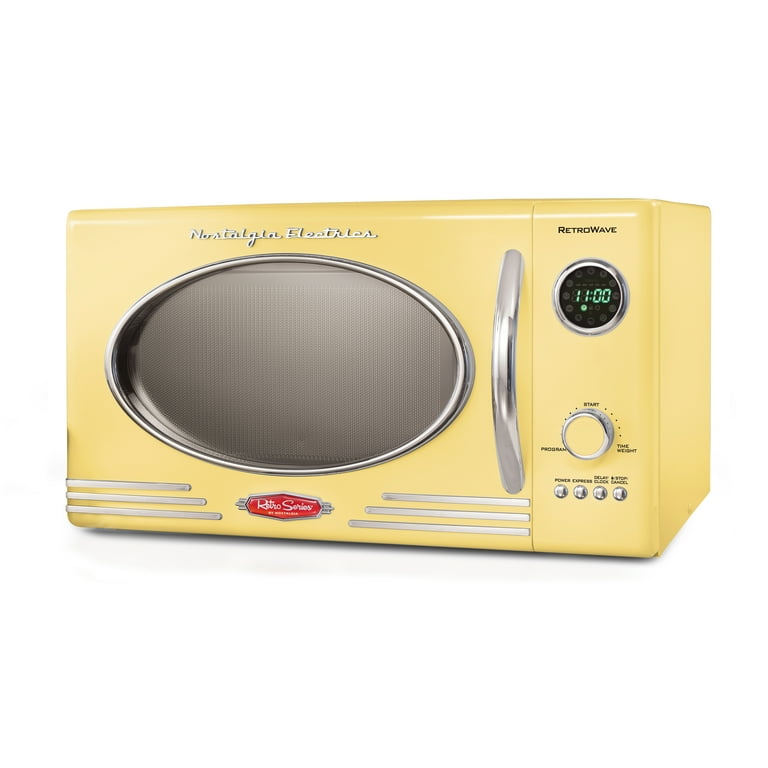This image showcases a retro-inspired microwave in a distinctive mustard yellow hue, reminiscent of the 1950s or 1960s. Positioned against a white background, the microwave features an array of nostalgic details. Above the large oval viewing port, which has a silver rim, is the text “Nostalgia Electrics” written in a classic font. This adds an authentic vintage touch to the design.

To the right of the viewing port, "Retrowave" is displayed in black text. Below this label is a circular digital display indicating the time as 11:00, with faint icons likely representing various settings. Beneath this display is a knob with a silver outline, and below the knob, there are four small silver buttons labeled (from left to right) as power, express, delay/clock, and cancel.

At the bottom center of the microwave, a red insignia reads "Retro Series." The front panel also features three horizontal lines on either side of the viewing port, further emphasizing its retro aesthetic. A chrome handle is situated to the left of the control elements, complementing the overall vintage design of the appliance.